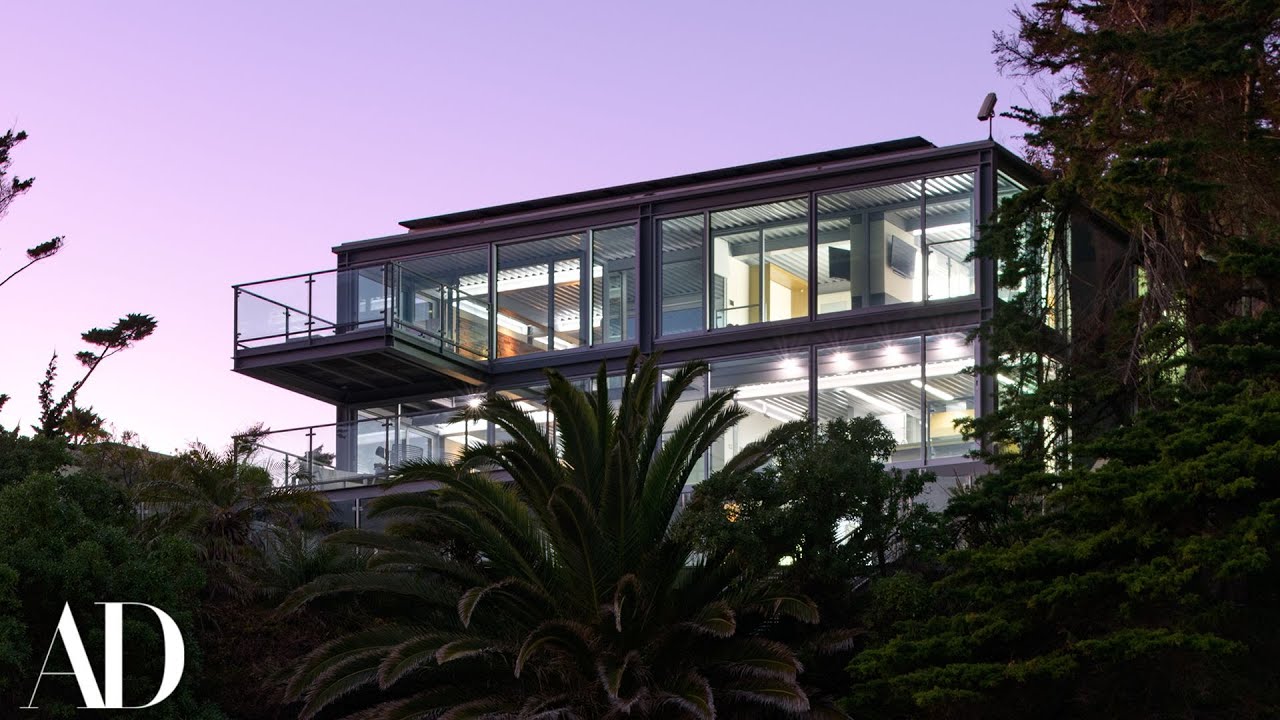The photograph captures a strikingly modern building, likely from a magazine, as indicated by the "AD" in prominent white font at the bottom left, suggesting it could be from Architectural Digest. The building itself is almost entirely glass with sleek metal frames, providing an open and airy feel. It appears to be a two-story structure, perhaps an office or a large contemporary residence, with two balconies—one on each floor—situated on the left edge of the picture. These balconies feature glass barriers and extend outward, enhancing the building's modern aesthetic. The ceilings inside are gray with distinct lines running across them. The sky above the building is a serene light purple, adding to the picturesque quality of the scene. Surrounding the building, there is abundant greenery, including trees and various plants that frame the image from the right side and partially from the left and bottom edges. A camera is visible on the top right corner of the building, directed downwards, adding a subtle detail that complements the overall sleek and secure design.